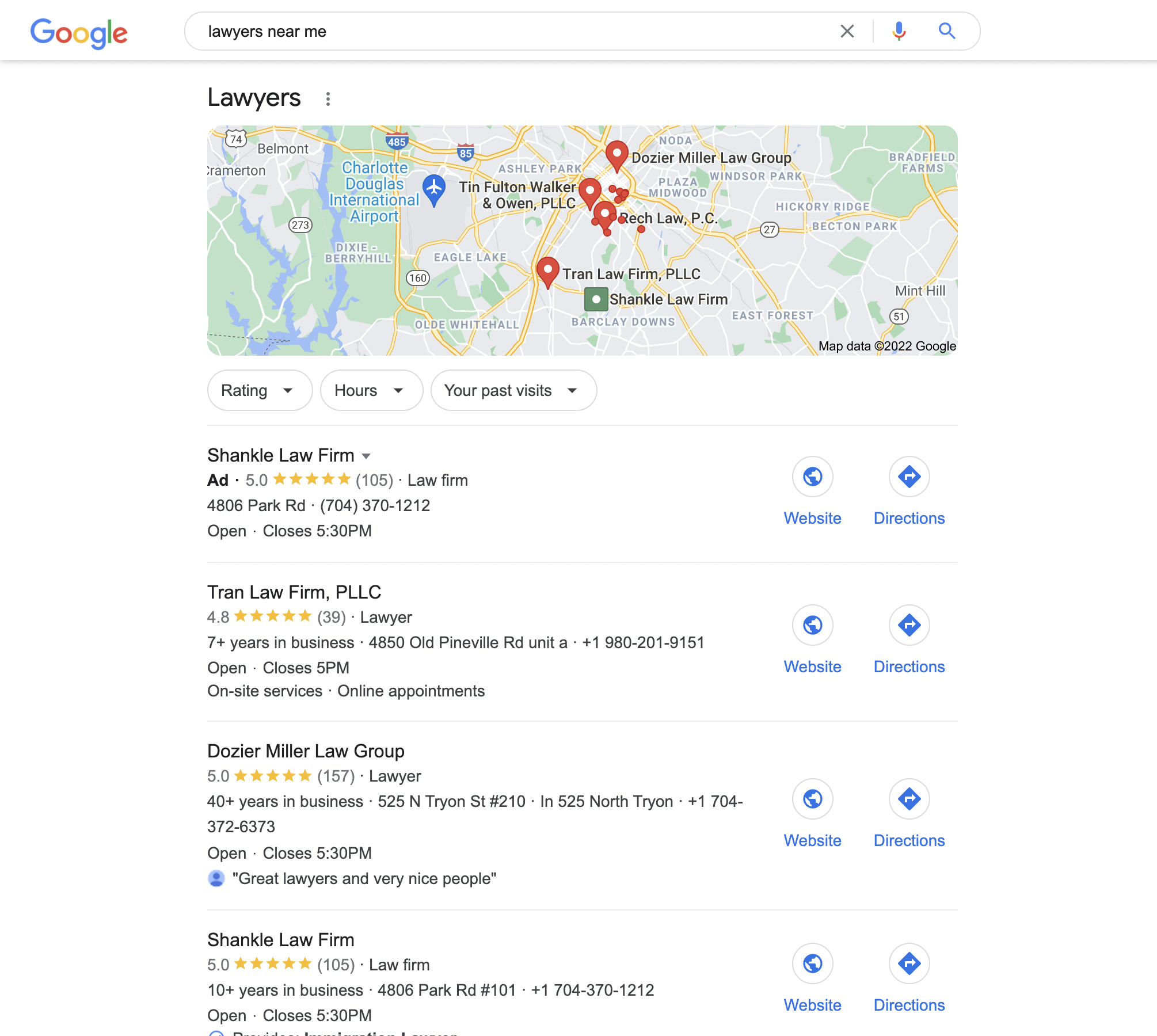This screenshot from a Google search displays a detailed query for "lawyers near me." In the top left corner, the familiar Google logo is visible, followed by the search box containing the query. Directly beneath the search box, the word "lawyers" is prominently displayed.

Below this text, a map of Charlotte is shown, highlighting various lawyer offices and firms throughout the city. Notably, Charlotte Douglas International Airport is marked on the map, confirming the city's identity.

Under the map, filtering options such as rating, hours, and past visits are available for refining the search results. The search returns a list of four law firms prominently displayed.

1. **Schenkel Law Firm** (marked as an ad) - This listing has a perfect five-star rating based on 105 reviews and is located at 4806 Park Road.
2. **Tran Law Firm, PLLC** - With a 4.8-star rating from 39 reviews, this firm is situated on Old Pineville Road.
3. **Dozier Miller Law Group** - This firm boasts a five-star rating from 157 reviews and is located at 525 North Tryon Street.
4. **Schenkel Law Firm** (appearing again) - Reiterated information showing a five-star rating with 105 reviews.

This intricate display provides a comprehensive overview of the top-rated law firms in Charlotte, offering useful details to assist the user in their search for legal services.